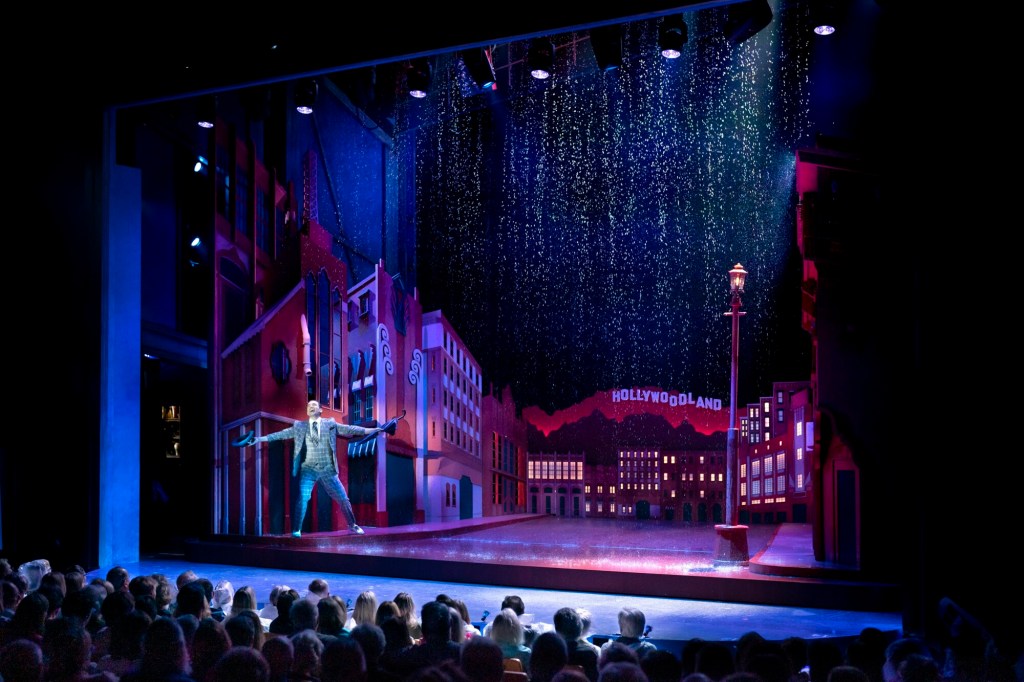The image captures a vibrant stage performance set in a darkened theater with at least four rows of an audience visible in the foreground. The performance takes place on a fairly small stage adorned with cityscape props, including a façade of high-rises and buildings that evoke an urban landscape. Dominating the background, a sign reads "Hollywood Land," mimicking the iconic Hollywood sign. Adding to the urban scenery, a street lamp stands to the right side, casting a soft glow. In the center of the scene, a man is performing, likely a rendition of "Singin' in the Rain." He's dressed in an older-style, checkered blue suit with a vest, dark tie, and possibly tennis shoes, accentuating the nostalgic feel. Holding a hat in his right hand and a dark umbrella in his left, he stands with his legs wide apart and arms outstretched, singing joyfully. Overhead, a pipe releases water, creating a rain effect that enhances the authenticity of his performance. The buildings in the backdrop, painted in dark hues of red and brown, some with illuminated windows, complement the nighttime city ambiance of the stage.